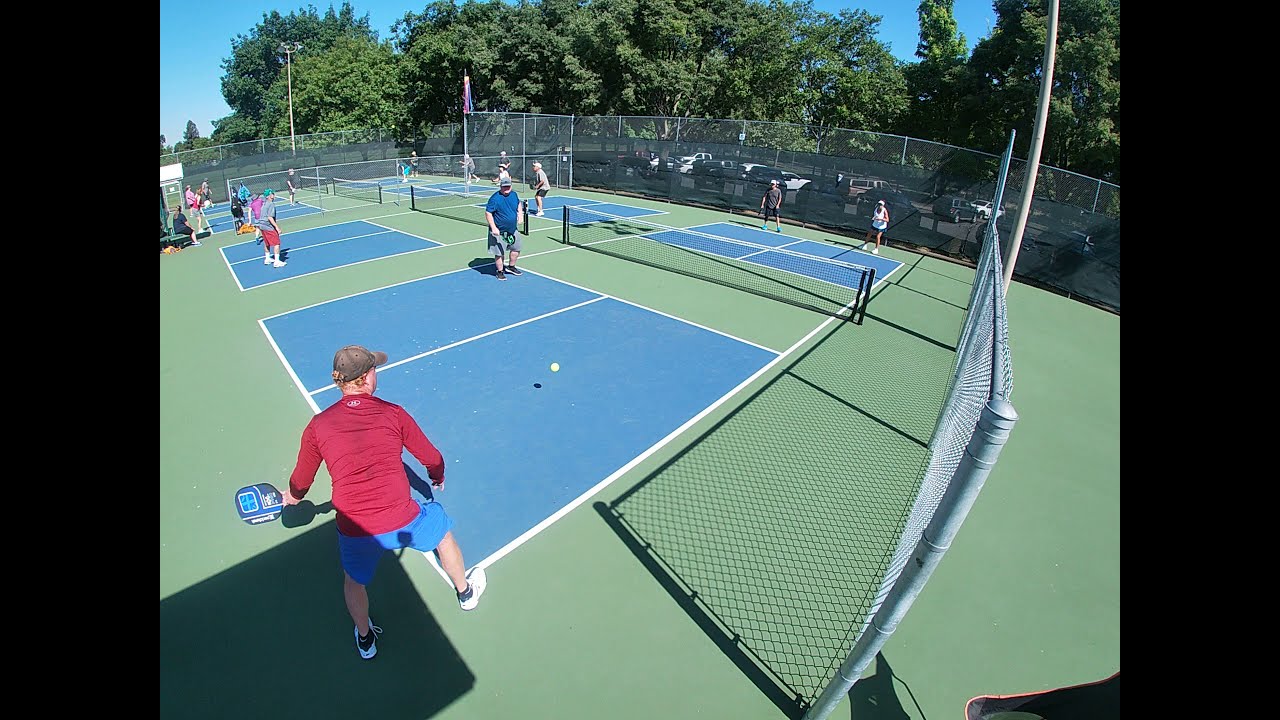The image depicts a dynamic outdoor scene of four pickleball courts aligned diagonally to the left. Each court features a blue playing surface, bisected by white lines, and enclosed by green turf close to the net. These nets are anchored by posts which vary in color from brown to black, and each net is topped with a white strip of fabric. Surrounding the entire court area is a tall, metal chain link fence, likely between 15 to 20 feet high. Players are engaged in active games on all courts, with typically two players per side.

In the closest court, a male player clad in a long-sleeved red shirt, blue shorts, and a brown hat is captured mid-action, holding a pickleball paddle. A yellow ball can be seen midair, just to the left of the image's center. Additional players, dressed in various sportswear, can be observed on adjacent courts, participating in doubles matches.

Beyond the fencing, the scene extends to a parking lot where several cars are parked. Encircling the parking lot is a green space filled with tall, lush, and bushy trees that exhibit vibrant green leaves, enhancing the outdoor ambiance. Above the trees, the blue sky can be glimpsed, adding to the image’s overall serene and lively atmosphere.